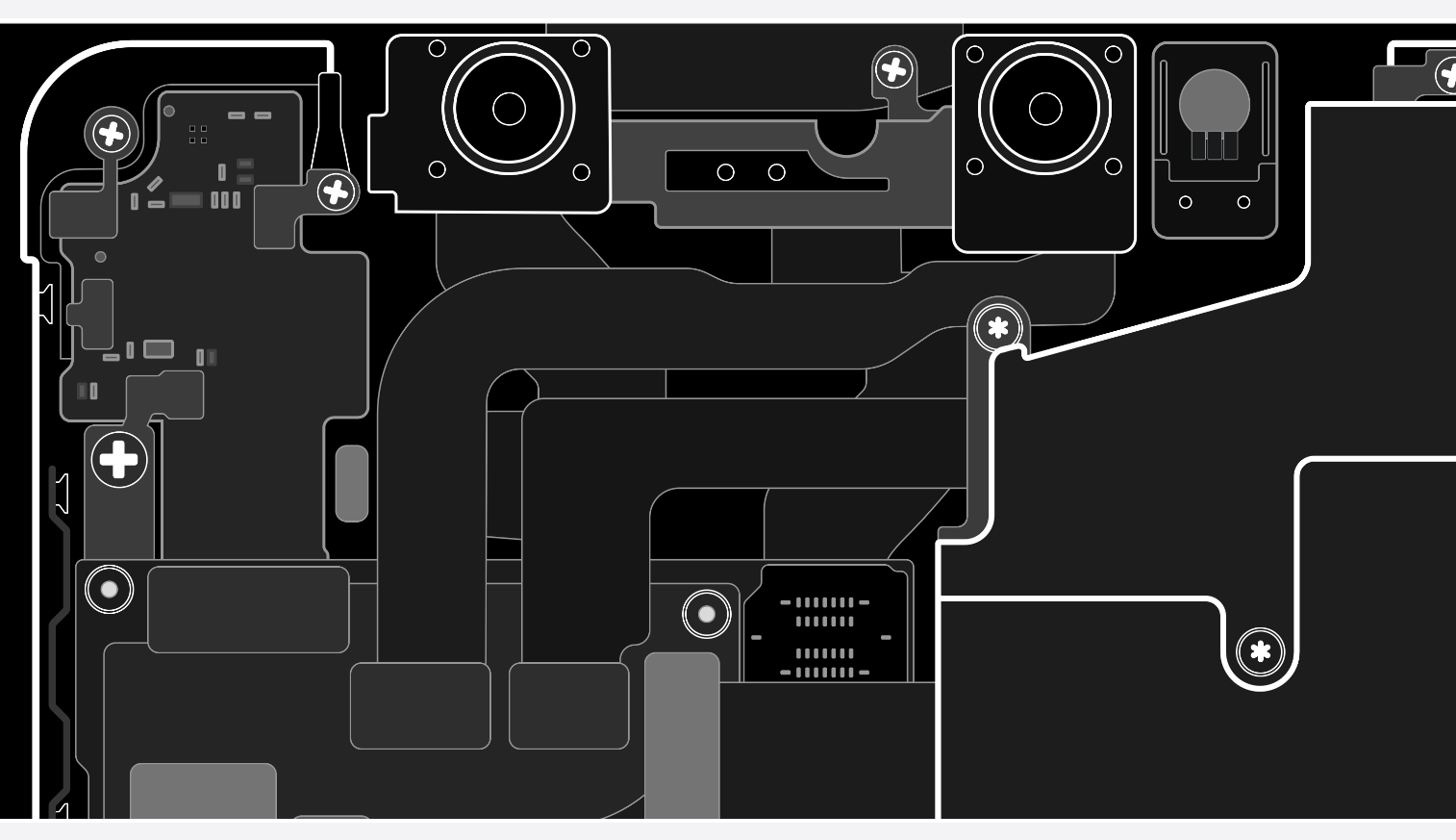The image appears to be a detailed, black and grayscale schematic design of the internal components of a laptop computer. At the top of the image, two squares resembling fans are evident, each with circular designs likely indicating the fan structures. To the right of these fans, a rectangular insert is visible, which could represent a storage device. Scattered throughout the schematic are multiple small circles, some marked with plus signs, torque screw indicators, or simple circles, suggesting various screw placements for securing components. Various cables are seen interconnecting different parts of the design. At the bottom left, two thick cables connect to gray rectangles, possibly indicating the motherboard. The entire schematic, filled with various boxes, dials, and tiny components resembling storage boards or memory modules, seems to represent the intricate layout of a laptop's internal circuitry.